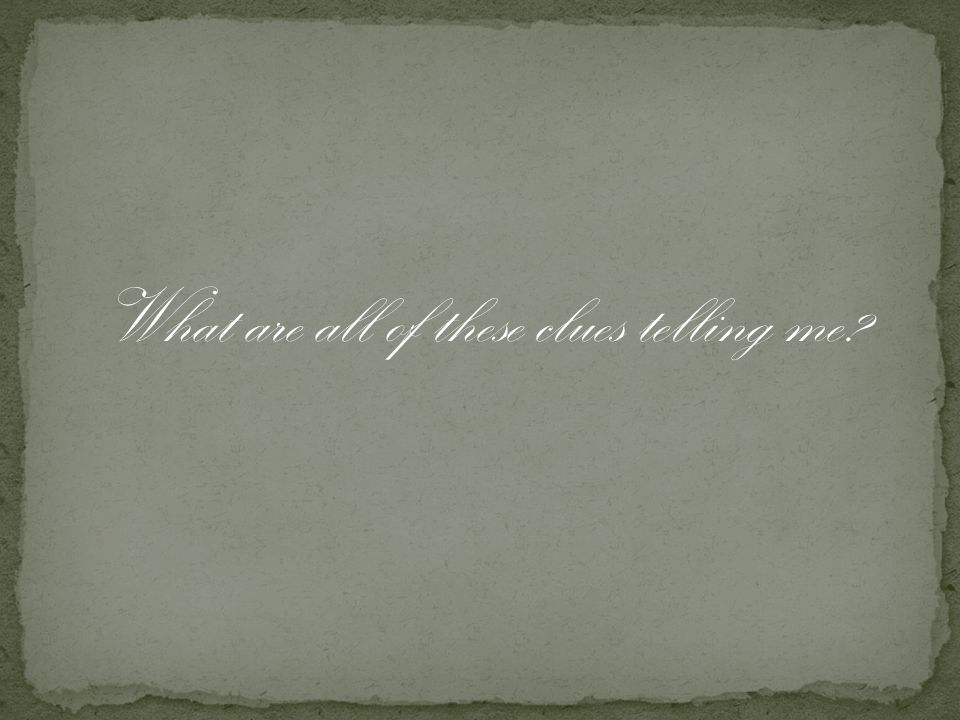The image depicts an elegant card with a light green background and a darker green border that appears slightly burnt or torched without any blackened effect, creating an uneven, dipped edge. The background itself is plain yet styled to resemble a weathered piece of paper with a few visible fibers, adding a touch of realism. Centrally displayed in a clean, italicized white cursive font are the words: "What are all of these clues telling me?" The text runs horizontally across the middle of the card, evoking the appearance of an intertitle from an old silent movie.